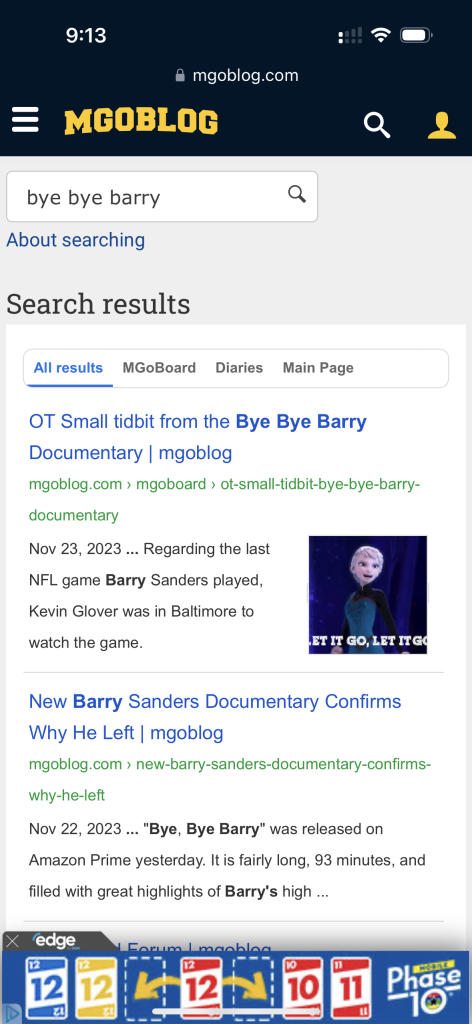The image depicts a webpage characterized by a black banner at the top. On the left side of this banner, the time is displayed as "9:13." Accompanying this, symbols indicate Wi-Fi strength, signal strength, and battery percentage. Directly below these icons is a lock symbol and the text "mgoblog.com" in small white letters.

Below the banner, three white lines are visible, followed by the large yellow letters "mgoblog." Adjacent to this is a search icon and a profile icon representing a person.

The next section contains a white box with the text "Bye Bye Barry," which is the search box, and underneath it, a blue link that reads "About Searching." Following this, the text "Search Results" appears in black, with four accompanying tabs. The first tab, labeled "All Results," is in blue and highlighted, while the next three tabs, "NGO Board," "Diaries," and "Main Page," are in black.

Further down, a title reads "OT Small Tidbit from the Bye Bye Barry documentary," followed by a horizontal line. The text "mgoblog, November 23rd, 2023, regarding the last NFL game Barry Sanders played" appears next, and to the right, a picture of Elsa with the caption "Let It Go, Let It Go." Finally, below this image, it reads "New Barry Sanders documentary confirms why he left MGO Blog."